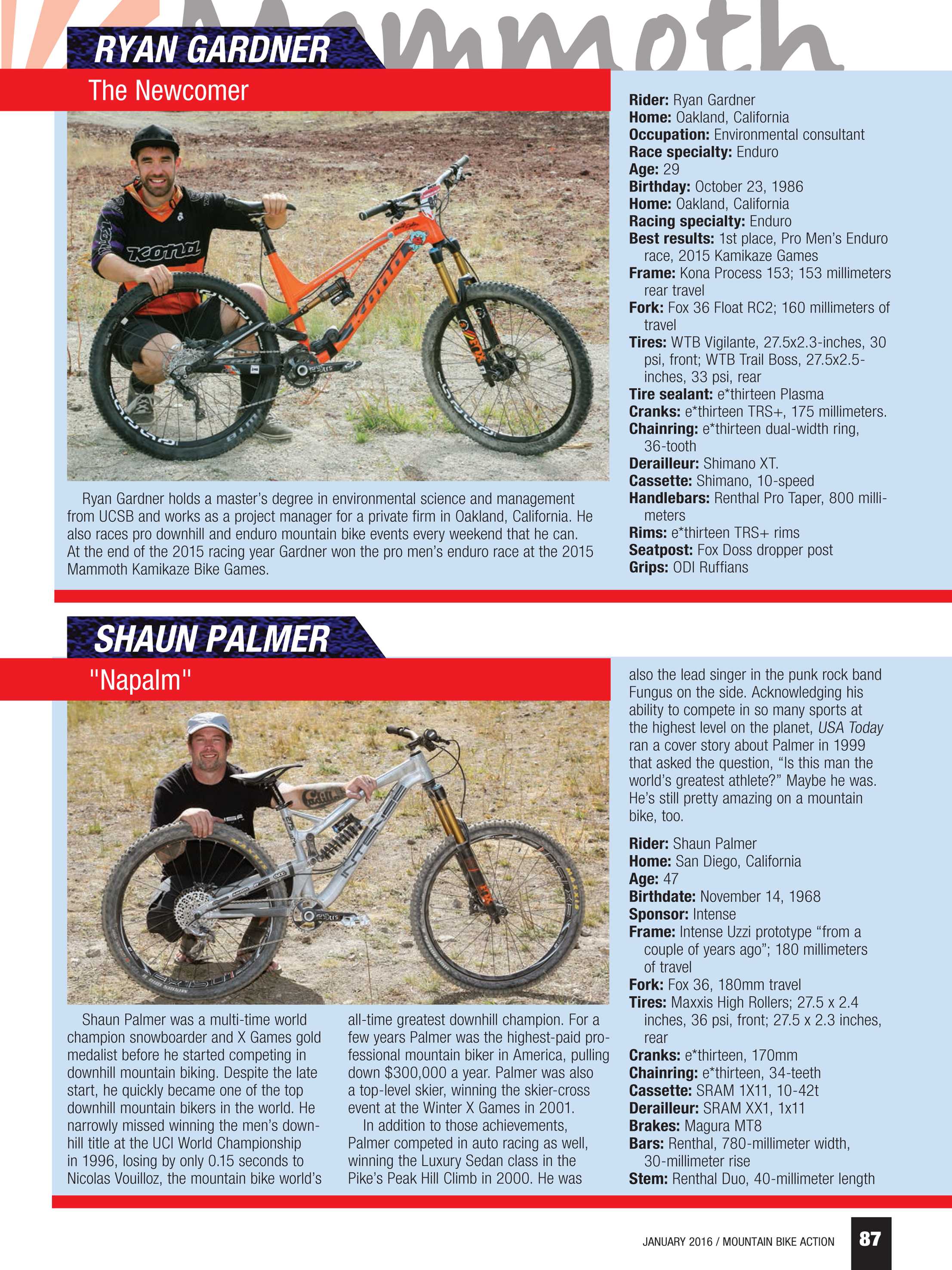This image is a page from the January 2016 issue of Mountain Bike Action, specifically page 87. It features profiles of two male mountain bikers: Ryan Gardner and Shaun Palmer. The top section highlights Ryan Gardner, dubbed "the newcomer." Ryan holds a Master's in Environmental Science and Management, and competes in both downhill and endurance mountain biking. His detailed statistics are listed on the right, including his age, birth date, and bike specifications. Ryan is in his 20s and hails from Oakland, California.

The bottom section profiles Shaun Palmer, nicknamed "Napalm." Shaun is an acclaimed multi-time world champion snowboarder and X Games gold medalist. Similar to Ryan, his age, birth date, and detailed bike information are provided on the right. Shaun is in his 40s and lives in San Diego, California. Each rider's profile includes a paragraph summarizing their background and achievements, along with a list of finer details such as their sponsors, bike frames, forks, and tires.